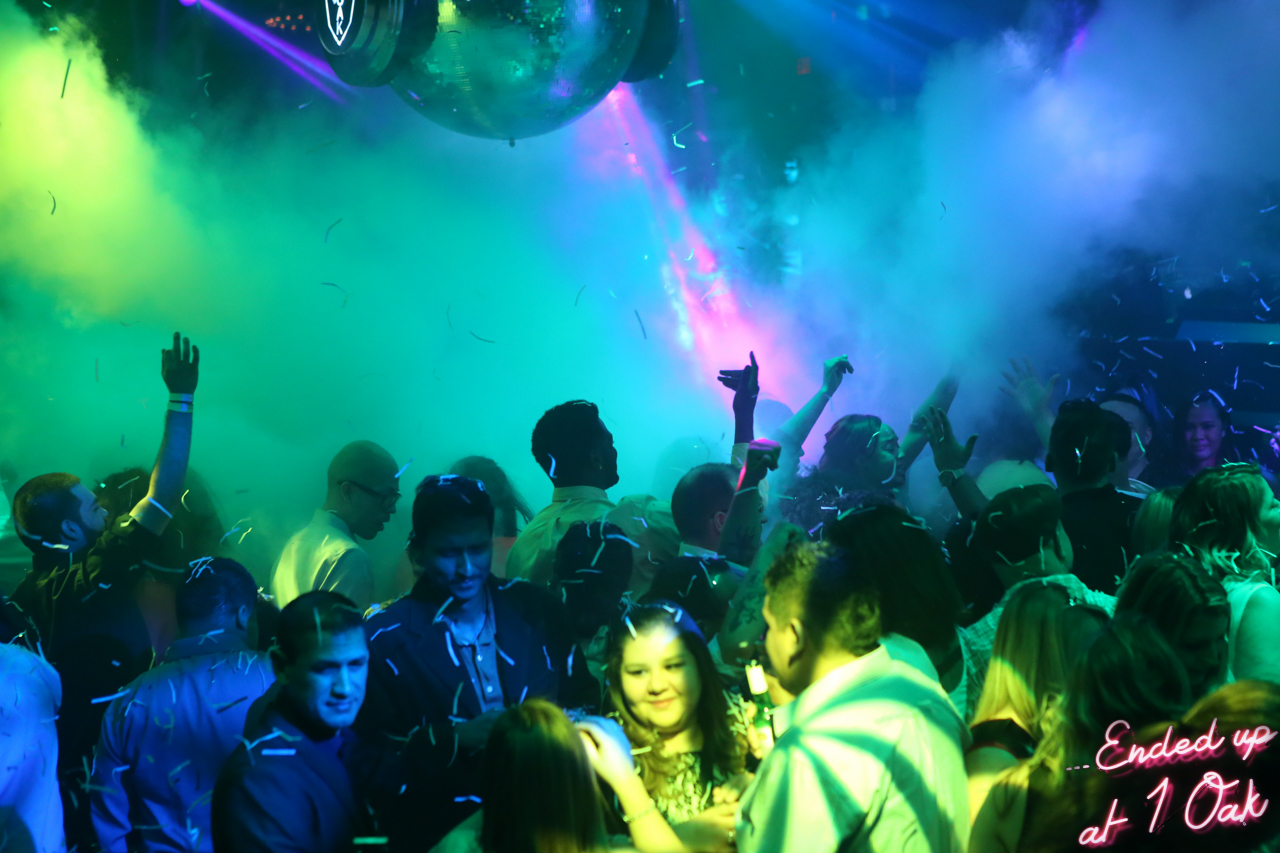The image captures the vibrant energy of a lively rave or festival. In the foreground, a diverse crowd of about 30 people of varying ages and ethnicities—including Hispanic, Asian, and white individuals—is seen dancing, talking, and mingling. They are covered in silver strands of confetti that are flying through the air. The room is suffused with atmospheric smoke and mist from multiple smoke machines in the background, creating an ethereal ambiance. Purple light rays project from the ceiling, adding to the colorful scene. Situated in the distance, several people are standing on a raised platform, barely visible through the haze. At the very top of the image, there is a round, bulbous machine that is currently inactive. In the bottom right corner, cursive pink text reads, "ended up at one oak." The scene is a cacophony of lights, colors, and joyous movement, perfectly capturing the essence of a bustling, popular festival.